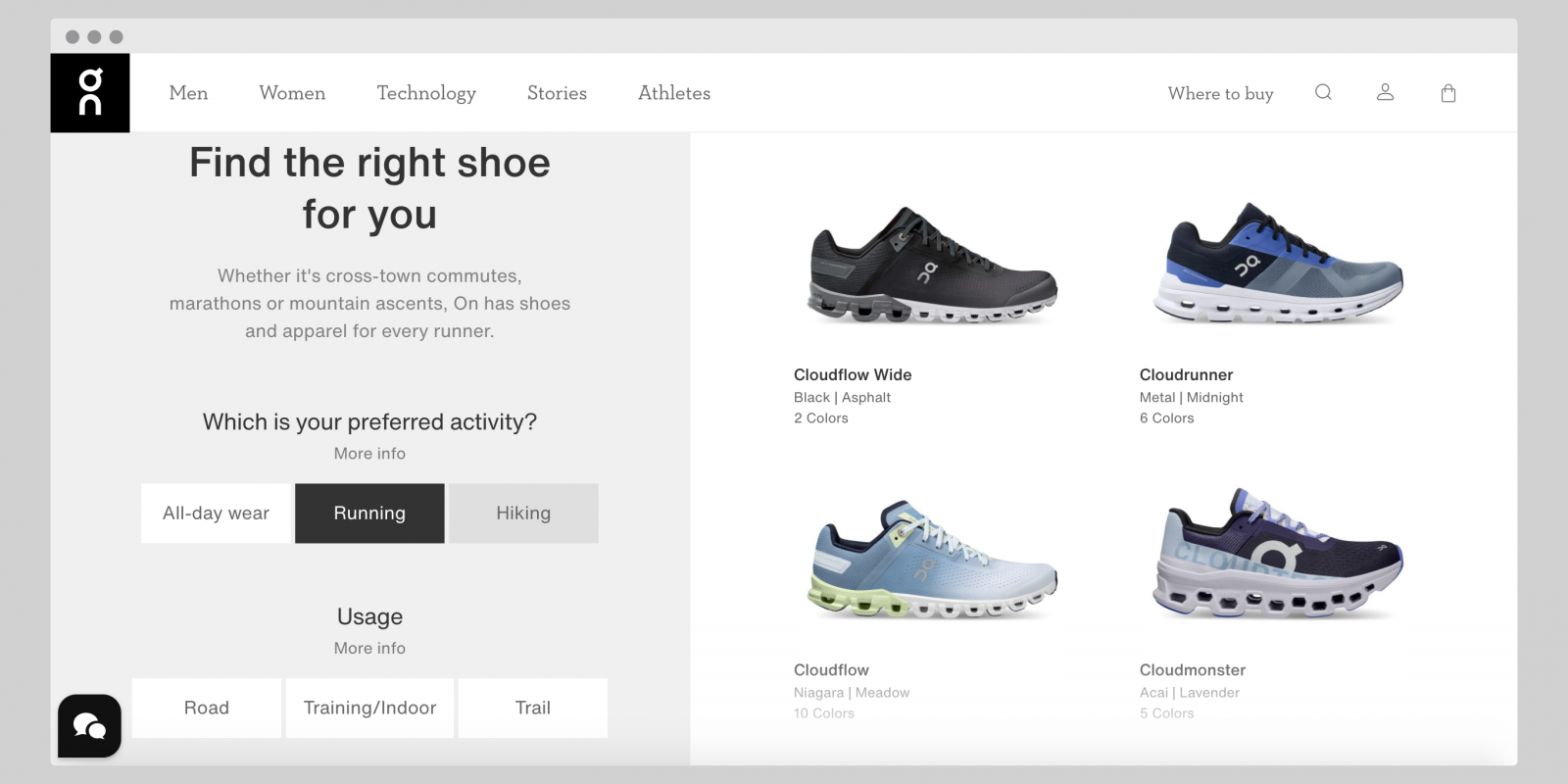The image depicts a sleek, modern website dedicated to "Cloud Shoes," a brand of running shoes and trainers. The website features a minimalist design with a black background and a white logo positioned in the top left corner. The navigation bar at the top includes several categories: Men, Women, Technology, Stories, Athletes, Where to Buy, a search function, a profile icon, and a shopping basket icon.

On the left side, against a gray background, there is a prominent text section that reads: "Find the right shoe for you, whether it's crosstown commutes, marathons, or mountain ascents. On has shoes and apparel for every runner, which is your preferred activity." Underneath, users are given options to click on different categories: All Day Wear, Running, or Hiking. Further options for shoe usage include Road, Training, Indoor, or Trail.

In the main section, after selecting the Running category, four shoe options are displayed: Cloud Flow Wide, Cloud Runner, Cloud Flow, and Cloud Monster. The image captures the website's clean and user-friendly design, emphasizing its functional categorization to help users find the perfect shoe for their specific running needs.